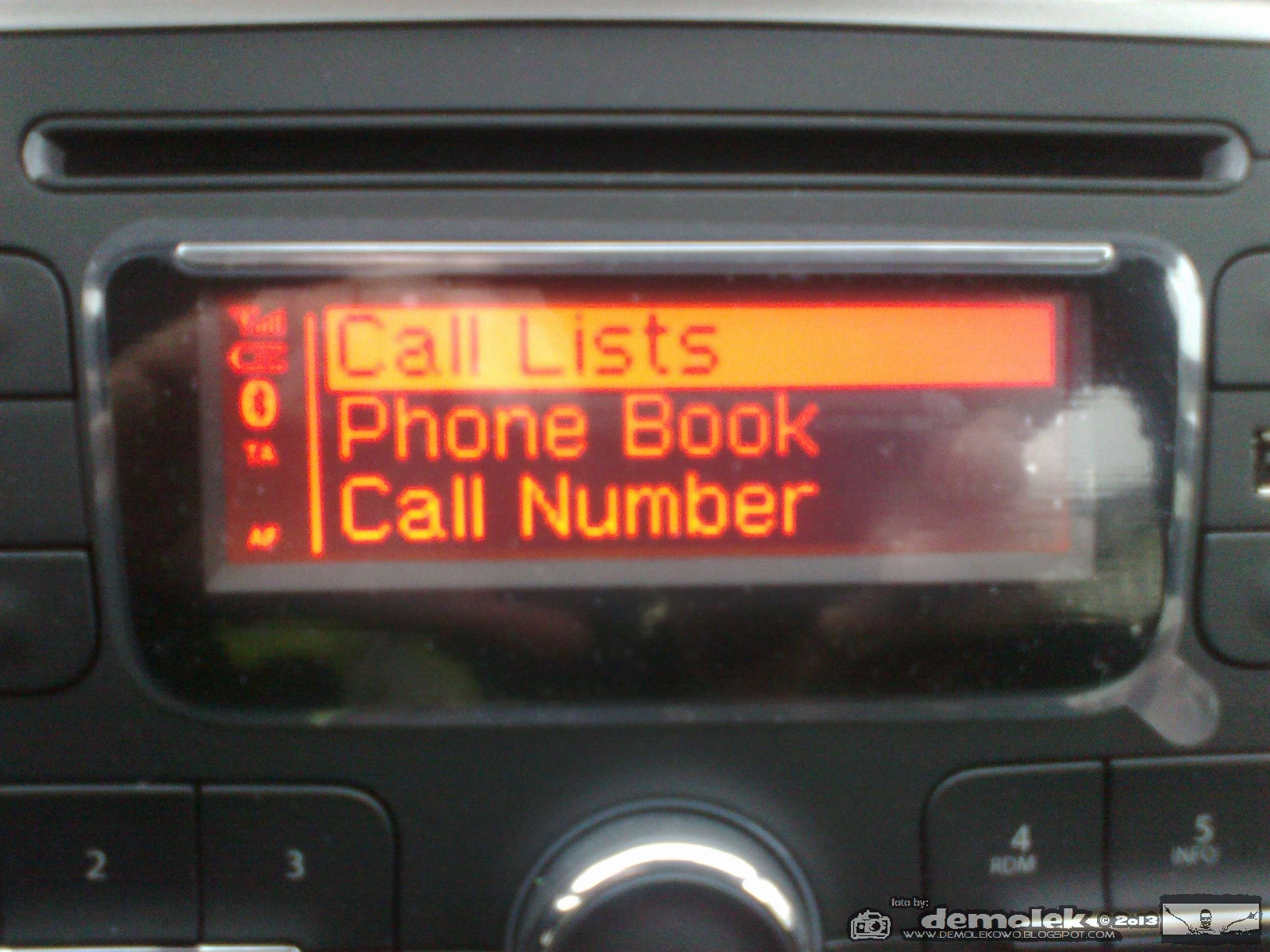This photograph captures the center console of a vehicle's radio system, showcasing a detailed view of the display screen and surrounding controls. The screen prominently displays three options in orange text: "call list" (highlighted with a contrasting black background), "phone book," and "call number." The area surrounding the display screen and buttons is a dark grey or black color, featuring additional symbols and buttons on either side of the screen. Below the screen, there is a circular knob and numerical buttons labeled "2," "3," "4," and "5." The image also includes a watermark in the bottom right corner, which appears to read "Demo-Lac" or a variation thereof, suggesting some form of placeholder or demo label. The screen still retains its protective peel-off tape, giving the unit a new or barely-used appearance. Additionally, a battery indicator symbol is visible on the left side of the screen, further detailing the car's audio system functionalities. The overall design and components suggest that this radio system is from a vehicle manufactured in the early 2000s to early 2010s.